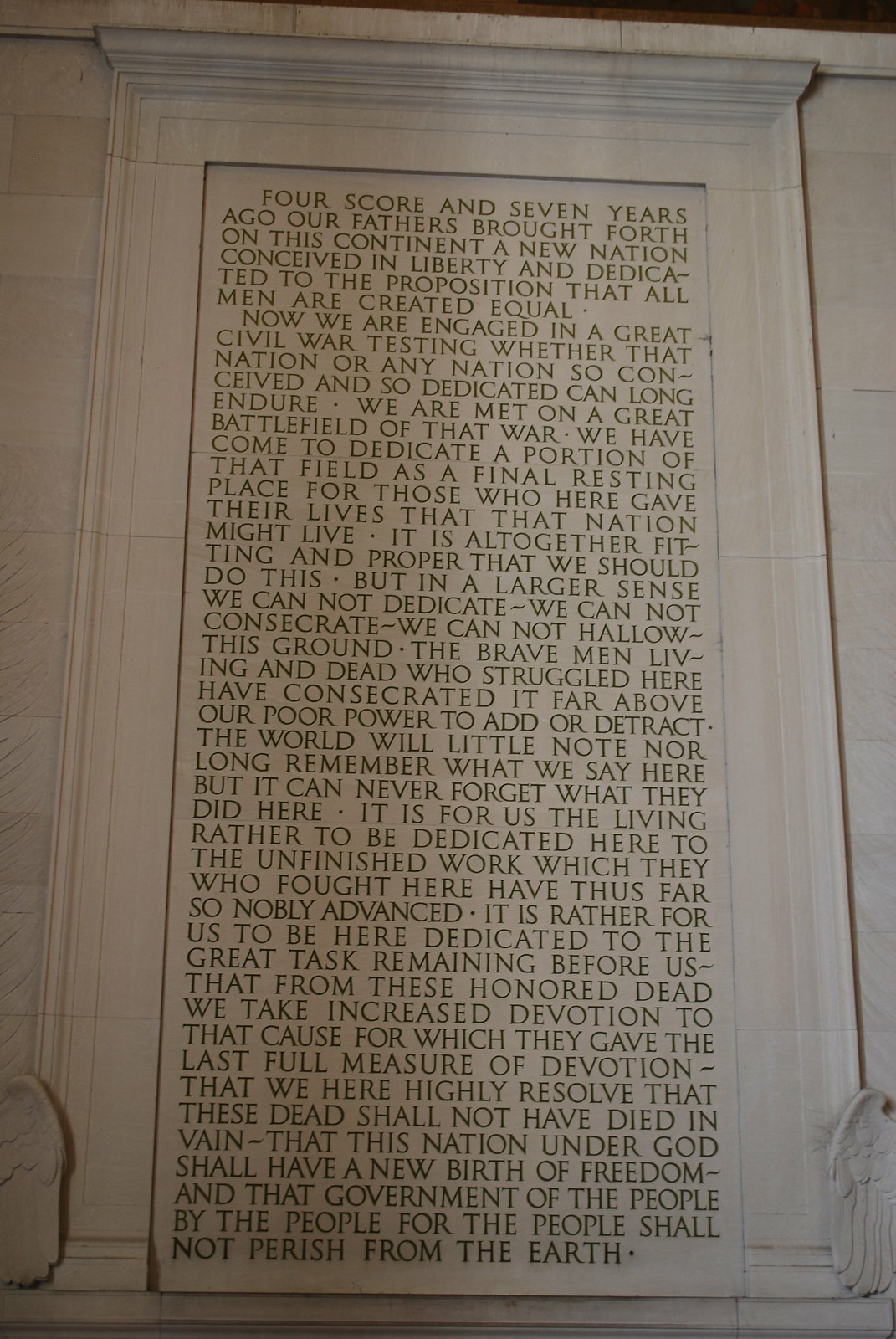This photograph captures the interior of the Lincoln Memorial in Washington, D.C., focusing on a large, white marble wall inscribed with the text of the Gettysburg Address. The stone wall, which appears the size of a standard door, features the iconic speech from President Abraham Lincoln, starting with the renowned phrase, "Four score and seven years ago." The inscription is elegantly framed within an archway and is meticulously engraved with capitalized letters that stretch across approximately 30 lines. At the base of the wall, there are two half-visible eagle wings, adding a touch of artistic detail to the solemn and historical monument. The wall's top has rounded parts, complementing the overall historic and architectural design dedicated to honoring the memory of those who sacrificed their lives in the Civil War.